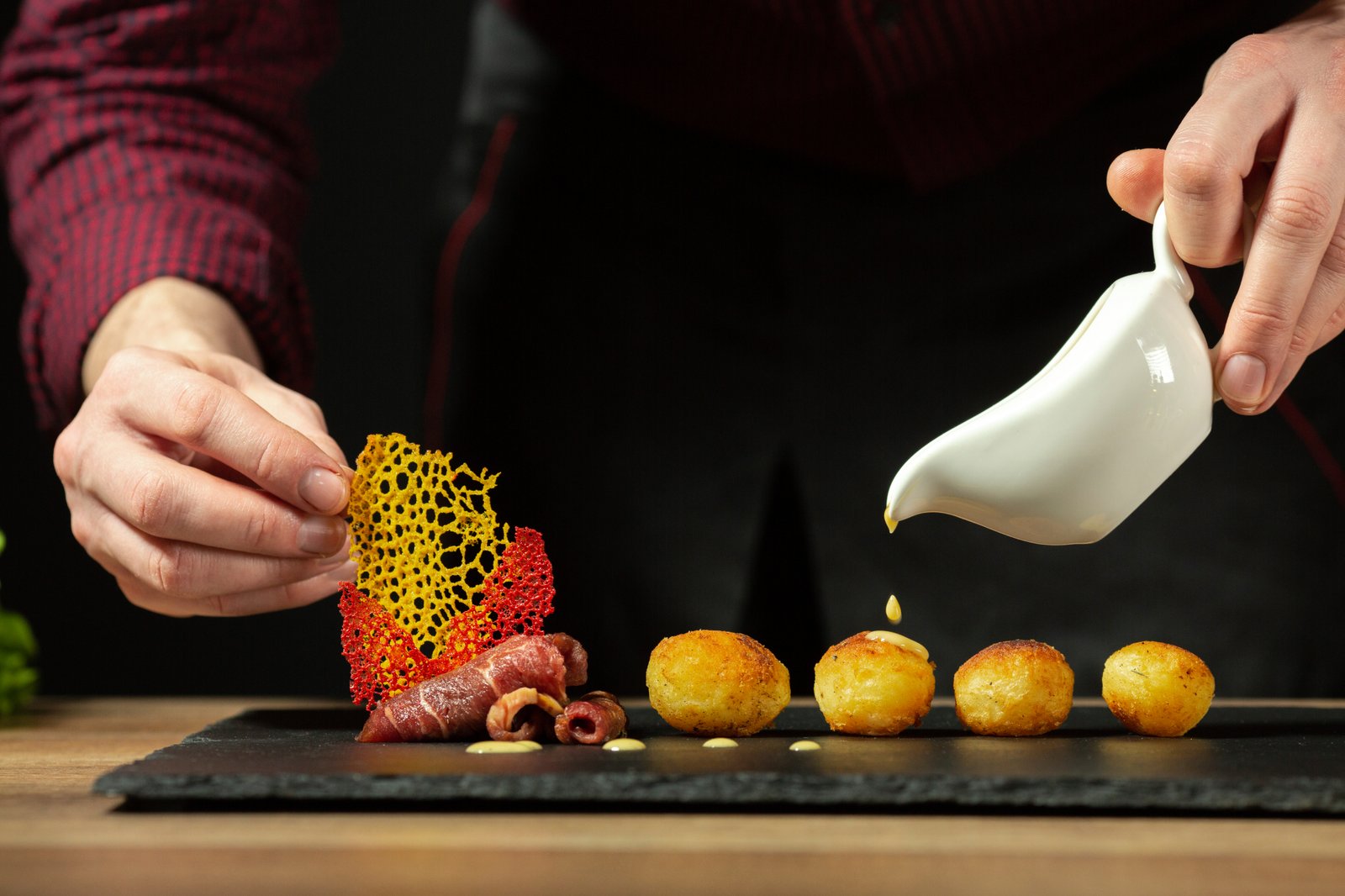In the color photograph, a close-up captures a Caucasian person meticulously preparing food on a black stone slab resting on a wooden countertop. The individual, wearing a long-sleeve red and black checkered shirt along with a black apron, is handling culinary elements with precision. You can see only their hands: the left hand holds a white gravy boat or sauce dish, dripping a yellow topping—possibly cheese or a cream sauce—onto a row of four round, fried pastries or cheese puffs arranged from left to right. These light brown puffs appear to be similar to hush puppies. On the black stone slab, to the left of the pastries, you see rolls of raw or cured meat, possibly bacon or steak tartare. Additionally, in their right hand, the person holds a red and yellow spongy, coral-shaped ingredient, potentially resembling deep-fried algae or seaweed. The countertop itself resembles a wooden cutting board. The overall setup suggests a highly decorative and detail-oriented culinary presentation.